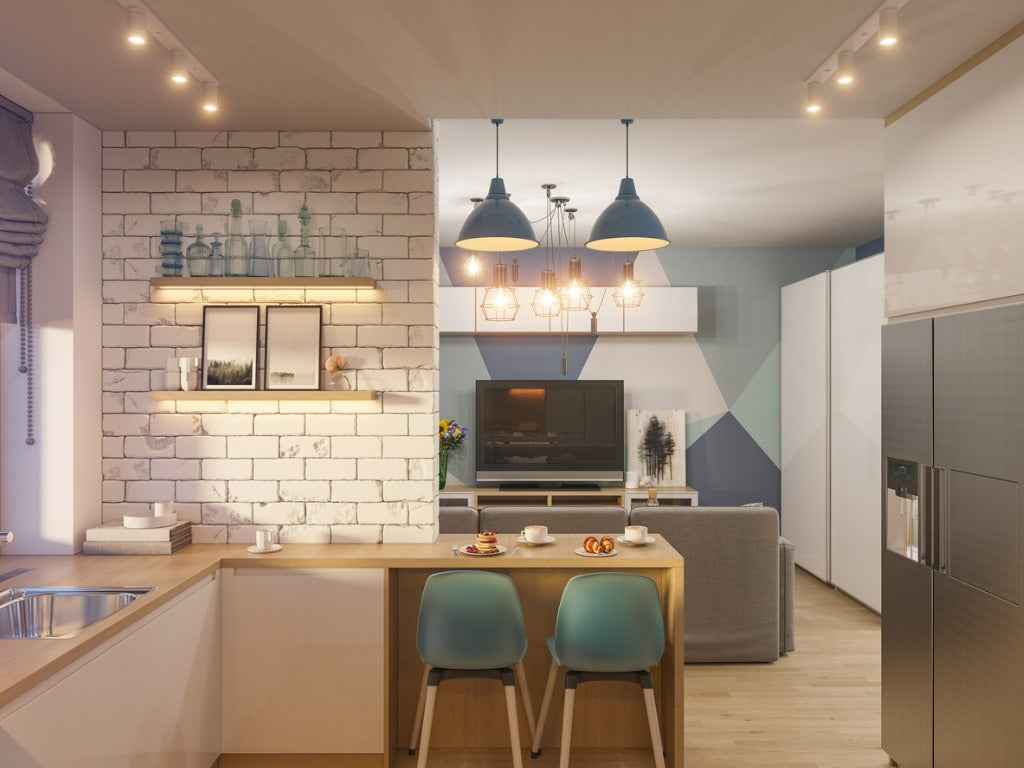The image depicts the inside of a well-lit, clean house, showcasing both a kitchen and a living room. In the foreground, the kitchen boasts a silver refrigerator with black handles situated on the right side. Adjacent to the refrigerator is a stretch of brown wooden countertop that features a silver sink on the left side and extends halfway across the image. On the corner of this countertop, against a white, brick-patterned wall, sit two stacked books. The brick wall spans from left to right and supports two shelves. The lower shelf holds two pictures and two flowers, while the upper shelf displays various glasses and bottles. Sunlight floods into the kitchen area, highlighting a breakfast setup with two blue chairs, two plates with muffins, and two cups of coffee.

In the background, the living room is visible. Its back wall features a geometric pattern in shades of blue, white, and light blue. A light gray couch, oriented towards a TV that sits on an entertainment stand, dominates the space. Adjacent to the TV, a vase with flowers resides on the left, and a painting of a forest hangs on the right. A white storage closet is positioned on the right side of the living room, and a chandelier with four lights illuminates the area. The entire space is well-lit with string lighting on the ceiling, enhancing the clean, organized atmosphere. The floors throughout the house are a beige-colored wood, contributing to the warm and inviting ambiance.